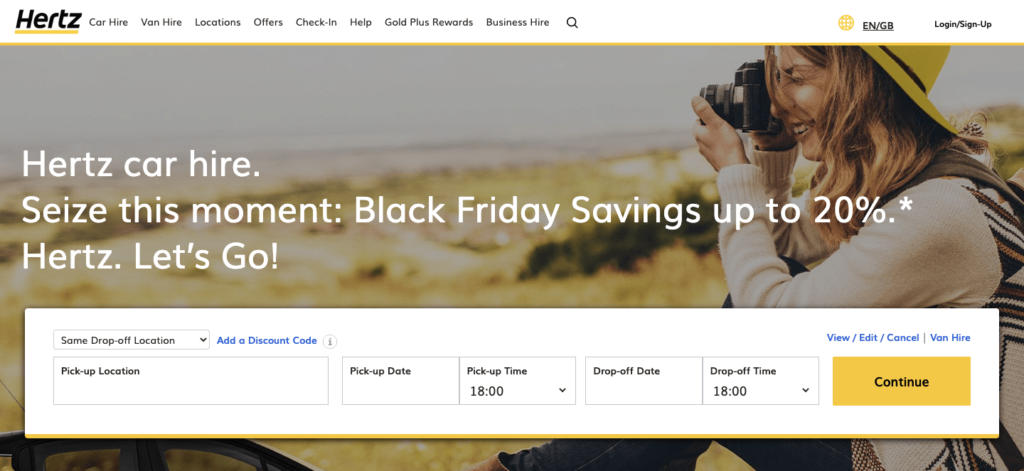The image depicts a webpage layout with a white header at the top, featuring the word "Hertz" in bold black letters with a yellow underline. The header includes a menu on the right side with options such as Car Hire, Van Hire, Locations, Offers, Check-ins, Help, Gold Plus Rewards, and Business Hire, along with a search icon. Adjacent to these options is a globe icon in gold color indicating language selection (EN/GB), and log in/sign up buttons.

Below the header, the main section of the webpage showcases a vibrant image of a woman wearing a wide-brimmed yellow hat and a tan-colored sweater, looking to the left while taking a photo with a camera. Across the image, white text reads: "Hertz Car Hire - See This Moment - Black Friday Savings Up to 20% - Hertz Let's Go."

Underneath the promotional banner, there is a section for booking details with a checkbox for "same drop-off location" and a blue hyperlink to "add a discount code." Two text boxes are provided below for entering the pick-up location and pick-up date, respectively.